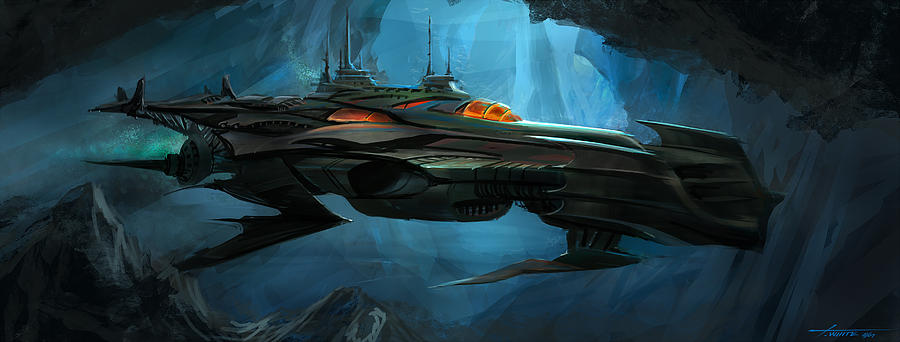In this evocative piece of digital concept art, a futuristic submarine navigates through an underwater cavern, not far from the ocean surface. Illuminated by beams of light streaming in from above, the scene is awash in shades of deep blue. The submarine, constructed from sleek metal and featuring a glowing red cockpit window, exudes a high-tech, sci-fi aesthetic. Its design is characterized by sharp angles and elements reminiscent of bat or dragon wings, particularly noticeable on its front and tail fin. Various antennas and equipment jut out from atop its hull, adding to its advanced, exploratory appearance. The submarine releases a trail of bubbles from its tail end, subtly indicating movement. Dark, cavernous surroundings envelop the vessel, juxtaposing the illuminated center and creating a mystical, almost otherworldly atmosphere that accentuates the submarine's glowing windows and the intricate, spire-like structures atop it.